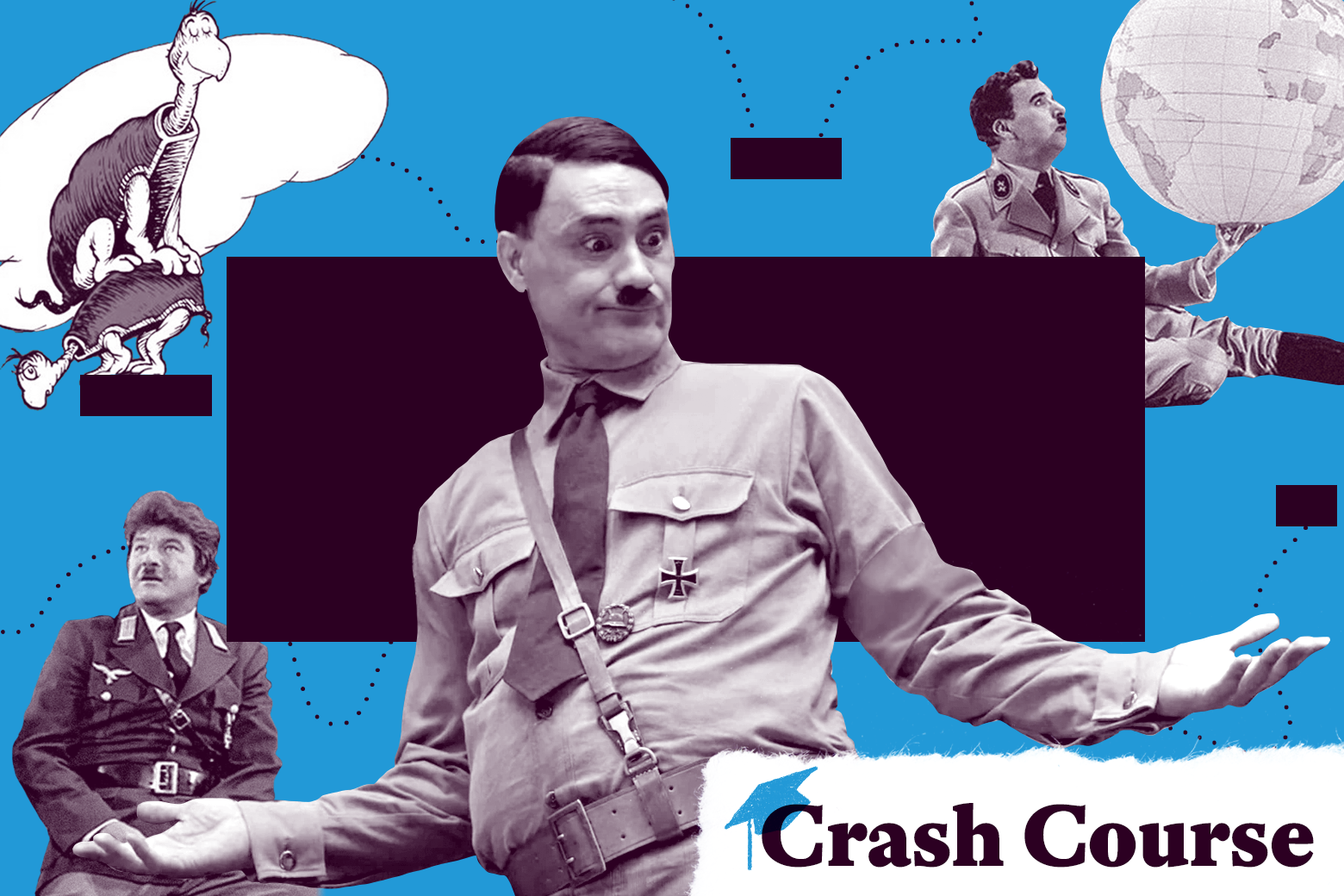In this detailed black-and-white image with a blue background labeled "Crash Course" at the bottom right, the central focus is a perplexed man dressed strikingly like Adolf Hitler. He sports the infamous short mustache and a combed, slick haircut characteristic of Hitler. Two other individuals, also mimicking this distinctive look with similar mustaches and period-appropriate clothing adorned with Nazi symbols, flank him. 

The man to the upper right, who has one boot kicked out in front, holds a globe resembling a balloon, injecting an air of surrealism. In the lower left quarter, another man gazes worriedly into the distance, adding a layer of anxiety to the composition.

In the upper left corner of the image, a whimsical touch appears with two cartoonish, Dr. Seuss-inspired turtles — one perched confidently on top of a concerned-looking companion, framed by a white cloud. A large black rectangle sits centrally behind the main figure, drawing further attention to his perplexed expression against the surreal and animated backdrop.